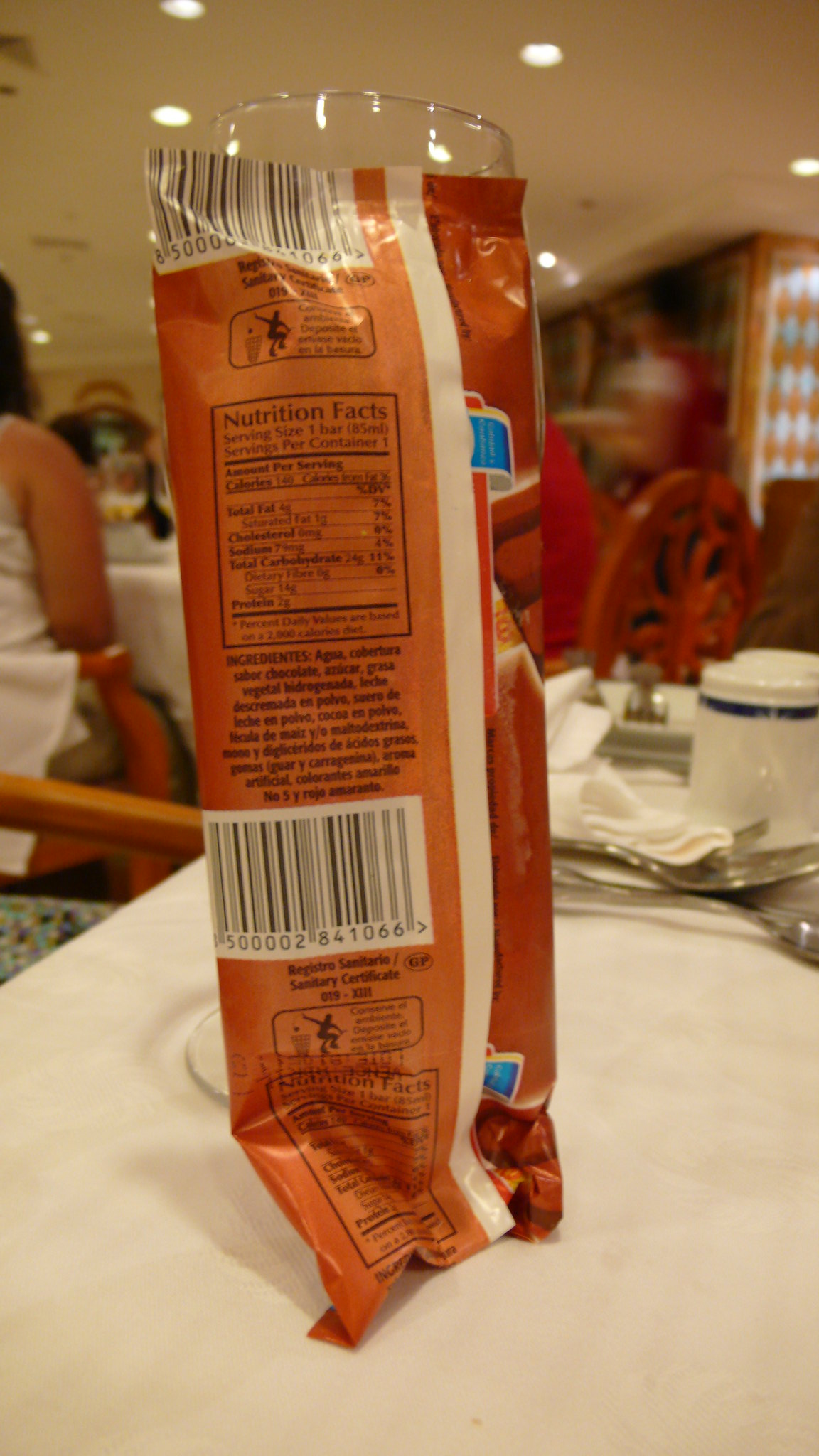This photograph prominently features a food package positioned against a wine glass at a restaurant setting. The food package is distinguished by an orange main body color and a black and white barcode near the top. Black font is partially visible, indicative of text wrapping around the other side of the package, and a blue ribbon-like design adds a touch of contrast. Beneath the nutritional information and ingredient list, another black and white barcode is present, followed by a secondary black nutrition label. The package rests on a white tablecloth, surrounded by silverware and white napkins, suggesting a formal dining environment. The background includes wooden chairs and other diners, contributing to the ambiance of an active restaurant.